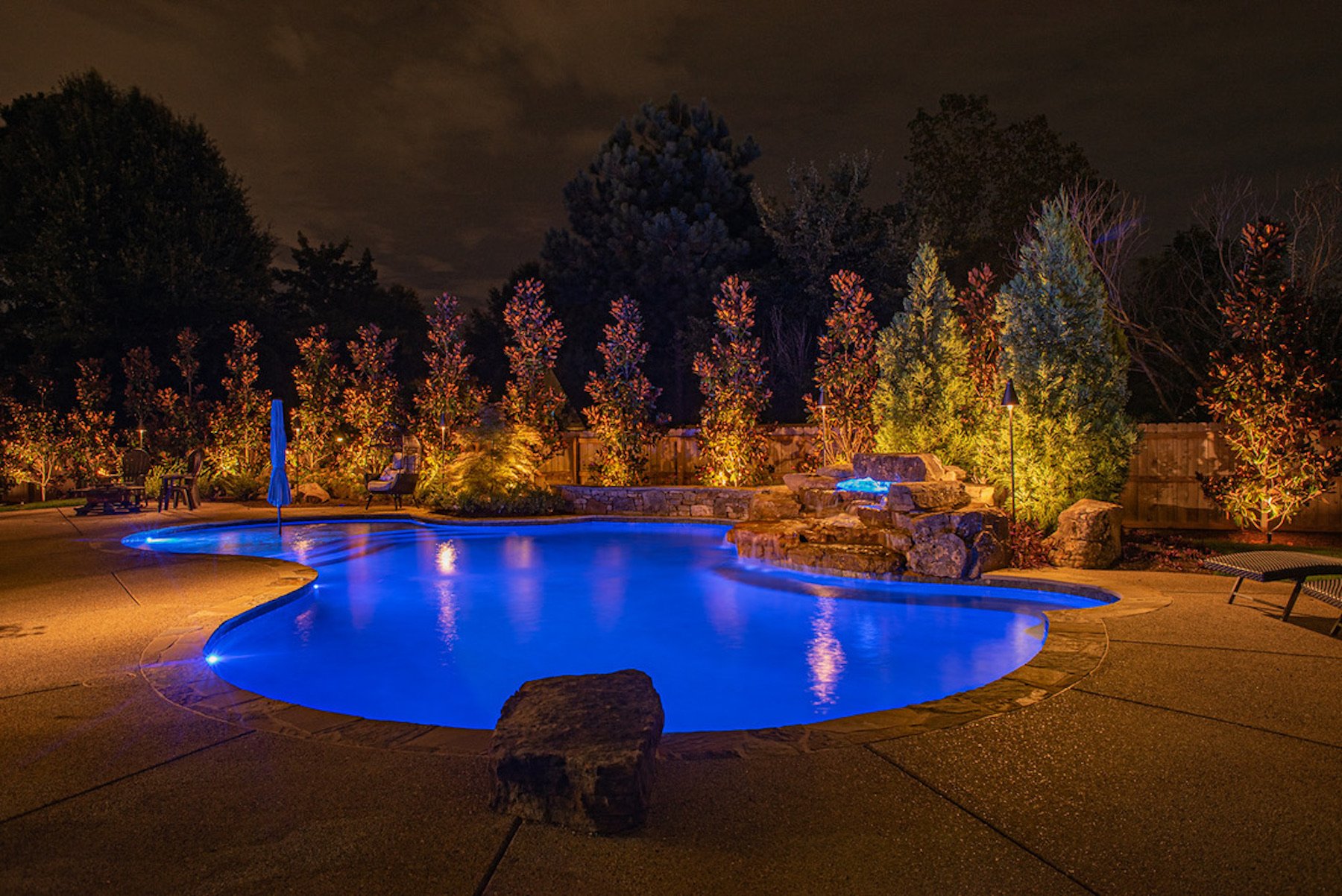The photograph captures a beautifully designed private backyard pool at night. The pool water, illuminated by underwater lights, appears as a striking crystal blue, creating a mesmerizing contrast against the darkening sky. The pool features an interesting shape, somewhat like a kidney with a semi-circular entry area, and includes a hot tub nestled into a bed of rocks, accessible via a set of steps. In the middle of the pool stands an umbrella, strategically placed to offer shade for a chair, though the area is currently unoccupied. Surrounding the clean and inviting pool are potted plants and a variety of trees and shrubs, contributing to a serene and secluded atmosphere. The backyard is predominantly concrete, bordered by a 30-inch stone fence, with freshly planted trees behind it, adding to the sense of a private retreat, likely situated in a forested area. The scene is devoid of any people or animals, enhancing the tranquil and pristine quality of this nighttime oasis.